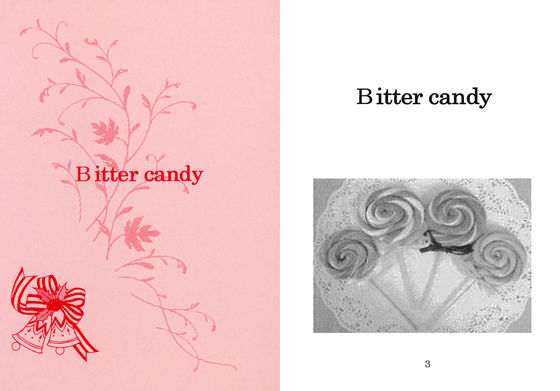The image consists of two distinct sections: the left section features a digitally created piece of stationery, while the right showcases a black-and-white photograph. The left side is a light pink rectangular shape with a slightly darker pink floral pattern, depicting branches with leaves and small flowers. In the middle of this rectangle, the bright red text reads "Bitter Candy." At the bottom left corner, there is an illustration of two bells tied together by a bow with a flower, also in red. 

The right side of the image presents a monochromatic photograph of four striped lollipops arranged in a fan pattern on a white lace doily. Above this black-and-white photo, the text "Bitter Candy" is written in black letters on a white background. Additionally, the number three appears underneath the lollipops. The positioning of the texts and objects aligns with their respective sections: the red text is almost centered in the pink rectangle on the left, and the black text is placed above the image on the right. The right section is notably smaller in size compared to the left.